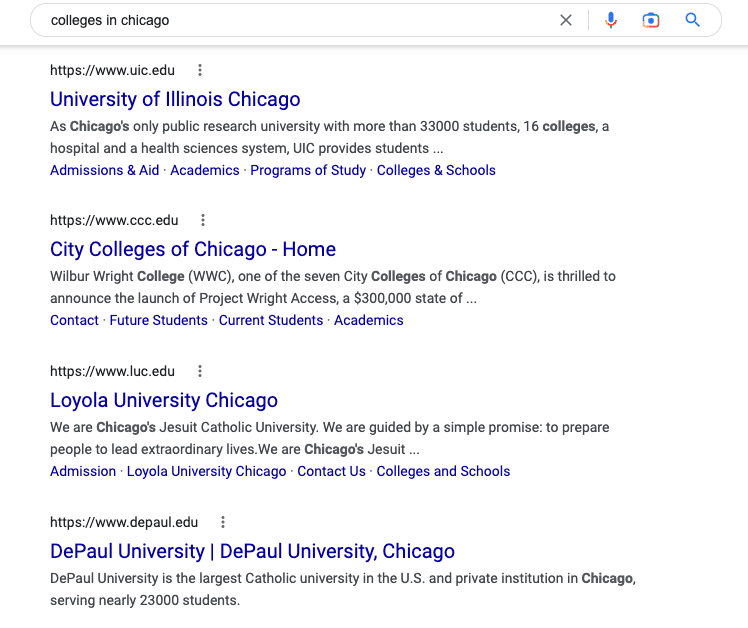This image is a detailed screenshot of a web search results page specifically for "colleges in Chicago." The background is predominantly white with no visible borders on the left, right, or bottom edges of the image. At the top of the page, there is a large search bar. Inside the search bar, the query "colleges in Chicago" is typed in black text. To the right of the search query are a gray X icon, a microphone icon, a square icon with a blue center, and a magnifying glass icon.

Below the search bar, four search results are prominently displayed. Each result is headed by a bold blue title, which includes "University of Illinois Chicago," "City Colleges of Chicago / Home," "Loyola University Chicago," and "DePaul University / DePaul University Chicago."

Directly above each title is the corresponding website address. Beneath each title, a brief description provides a concise overview of the respective institution, utilizing gray text and bold gray text for important highlights. 

At the bottom of each college listing, additional sections are available in clickable blue font. These sections include options such as "Admissions and Aid," "Academics," "Current Students," and "Contact Us," allowing users to navigate directly to the relevant parts of each college's website.